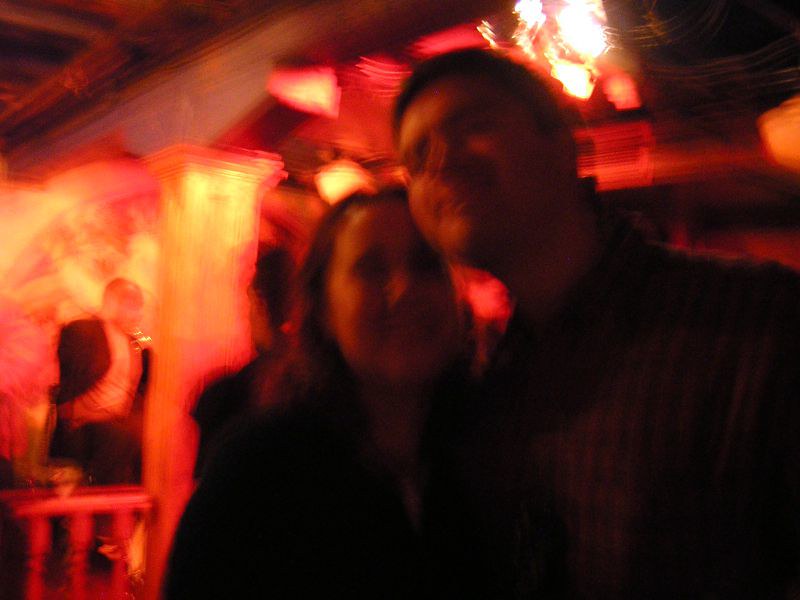In this somewhat unfocused color photograph, a couple is captured standing in the center of a dimly lit bar, with bright, warm-toned lighting that casts hues of red, orange, and yellow throughout the scene. The man, who is taller, leans in from the right, gently pressing his cheek against the forehead of the shorter woman, creating an intimate and affectionate moment. Their blurred faces suggest they are both smiling. They occupy about two-thirds of the image, which adds to the sense of closeness and intimacy. In the left-hand background, a shadowed figure of another man is faintly visible, adding depth to the scene. The foreground remains predominantly dark, in shadow, contrasting with the warm lighting around the couple. The photo appears to be a spontaneous snapshot, possibly a selfie or taken by someone unfamiliar with the camera settings, which resulted in an unfocused but heartfelt capture of the tender moment shared between the couple.